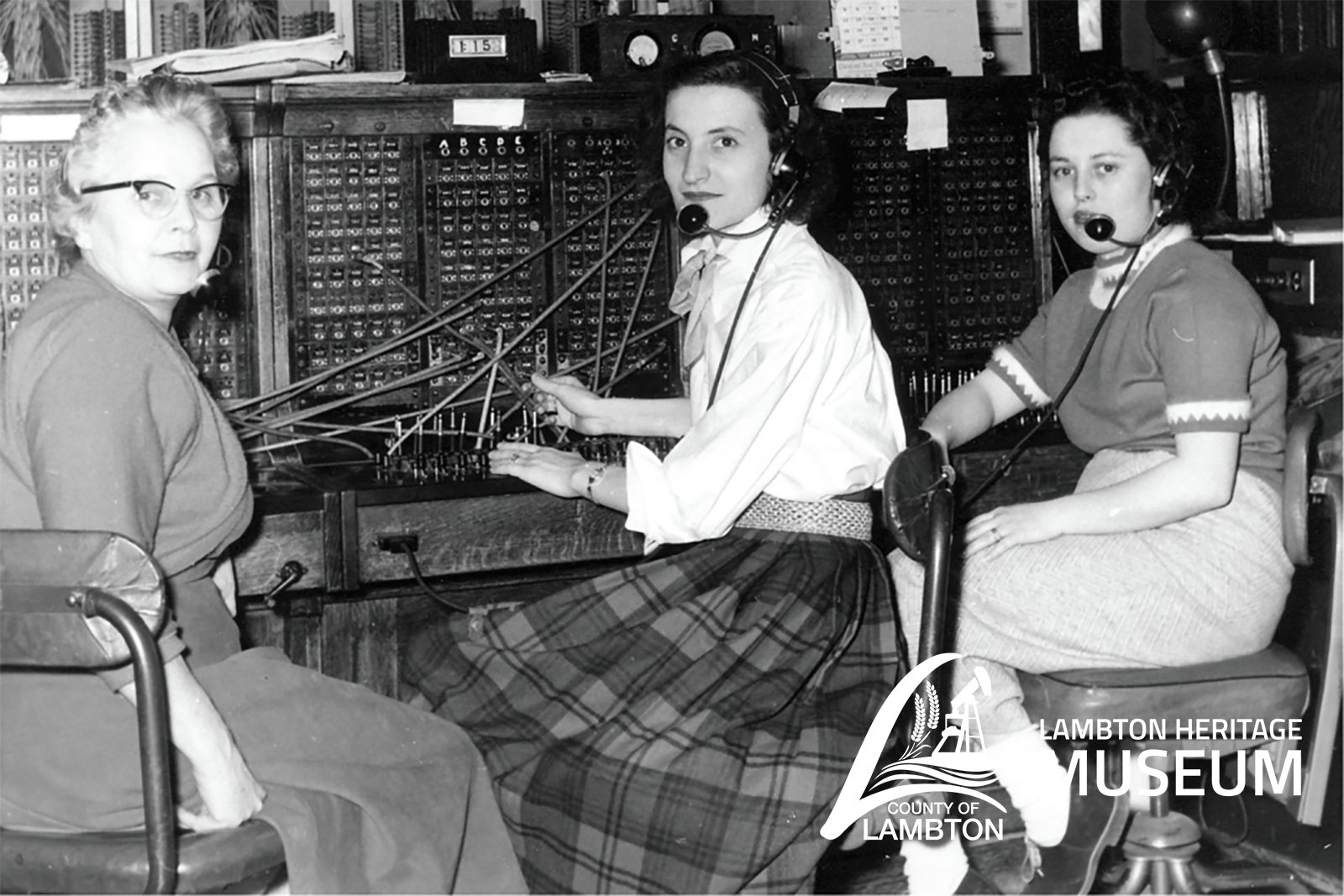This black and white photograph depicts three women, likely from the 1960s or 70s, positioned in a telecommunications setting. Seated at what appears to be a large switching station, they are all looking and smiling at the camera. Each woman is equipped with a headset featuring a microphone, indicating their roles as radio or communications operators. Their attire is modest and traditional for the era: 

- The woman on the left, notably older with glasses, wears a long-sleeved blouse paired with a checkered skirt.
- The woman in the middle, fairly young, is dressed in a long-sleeve shirt and a checkered skirt, and also has a headset on.
- The woman on the right is in pants and a buttoned-up short-sleeve shirt and likewise wears a headset.

Behind them, the work environment is filled with what appear to be server racks or computers, essential for their communications tasks. Notably, the bottom right corner of the image bears the inscription "Lambton Heritage Museum, County of Lambton," denoting its historical and regional significance.